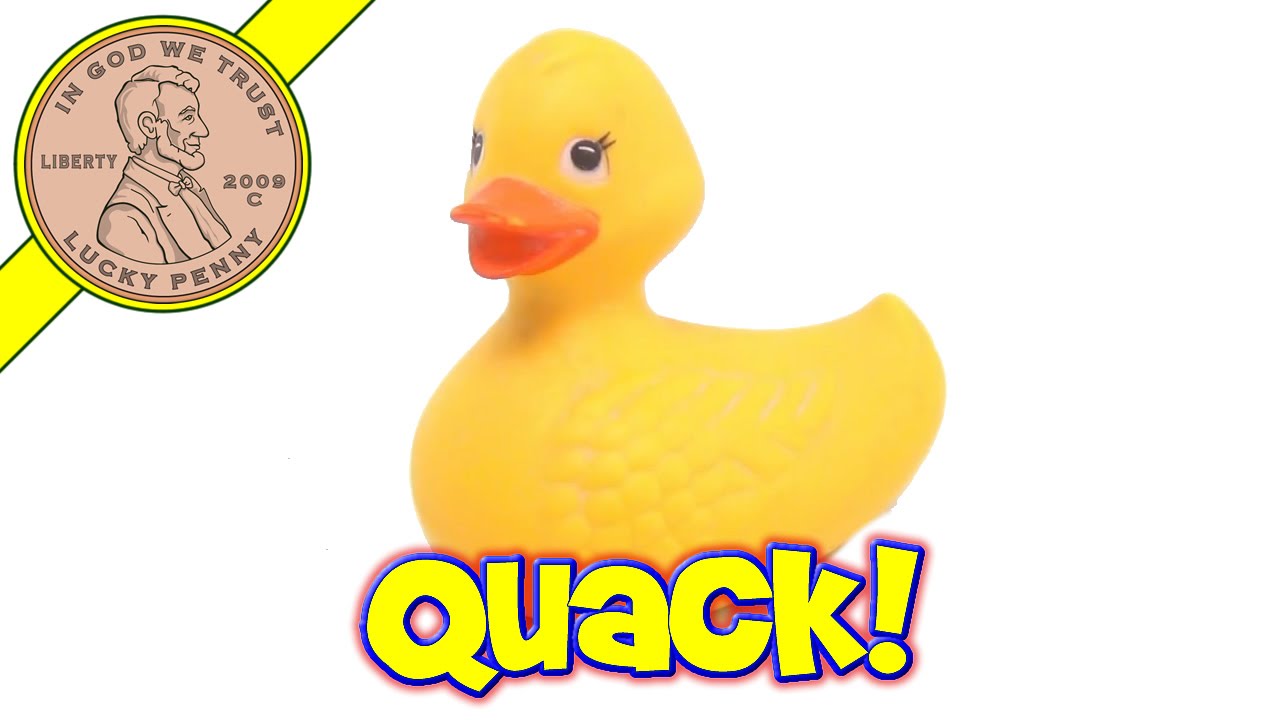The image features a yellow rubber duck, facing left, prominently placed in the center against a completely white background. The duck has an orange beak, white eyes, and distinctive black eyelashes, suggesting it might be a female duck. Detail on the duck includes a small textured area indicating a wing. Below the duck, in bold cartoony letters, the word "QUACK!" is written in yellow font outlined in blue with a slight red haze.

In the upper left of the image, there is an illustration of a penny within a yellow circular highlight, set against a diagonal yellow stripe that is outlined in black. The penny, showing Abraham Lincoln’s profile facing right, bears the text "In God We Trust" at the top, "Liberty" on the left, "2009 C" on the right, and "Lucky Penny" at the bottom, suggesting it’s a symbolic or novelty coin rather than an actual one. This combination of elements creates a whimsical, playful feel to the entire scene.